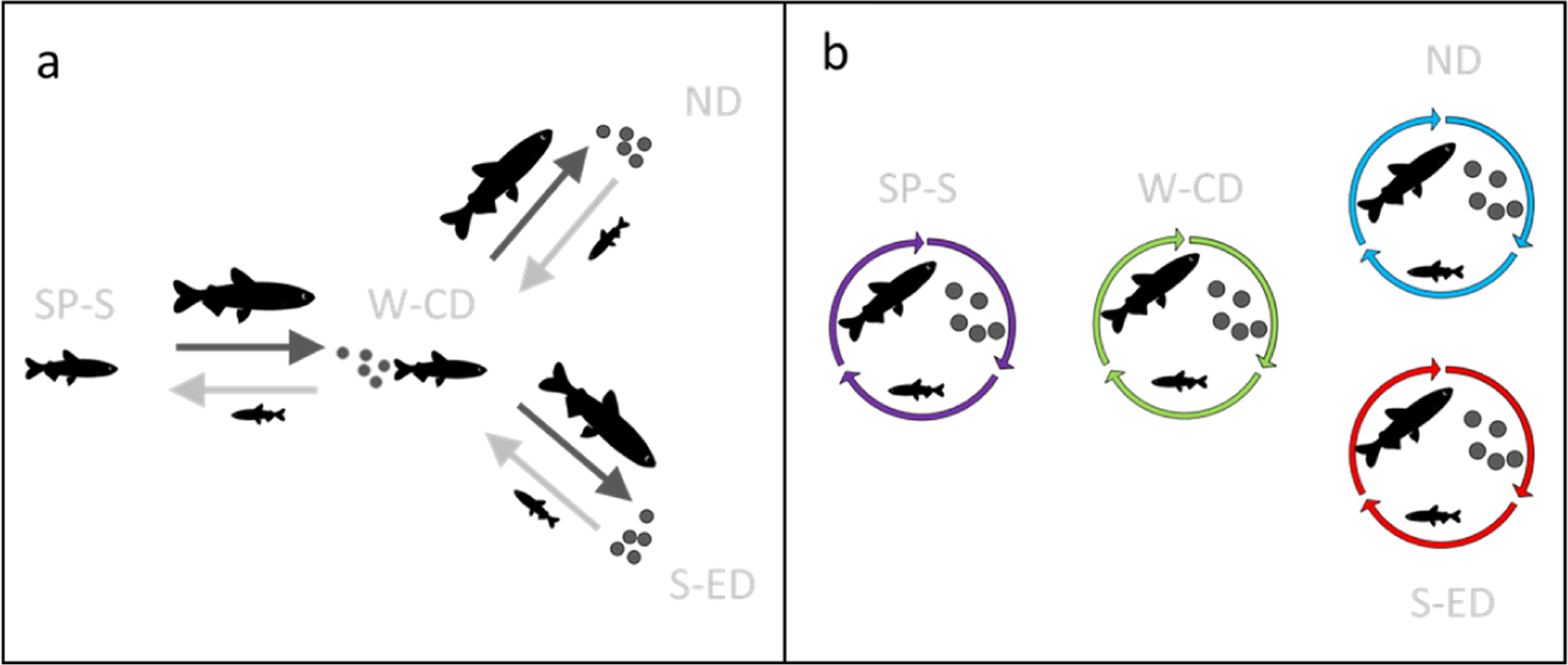The image features a detailed diagram split into two sections labeled A and B, both placed against a white background. In section A, on the left side, we see a black background with fish illustrations moving in various directions. The section is labeled with the terms SP-S, W-CD, ND, and SED. The fish are depicted swimming left to right and in multiple directions, indicating a potential life cycle or movement pattern. One fish is shown swimming towards the top right and another towards the bottom left, accompanied by arrows suggesting different paths.

In section B, on the right side, similar terms (SP-S, W-CD, ND, and SED) are used. This section features four circles colored purple, green, blue, and red. Each circle contains fish illustrations, with one fish facing upwards to the right and another facing left at the bottom of the circle. Additionally, there are five black dots within each circle, possibly representing eggs or another stage in the life cycle. Arrows within the circles suggest movement patterns or stages of development. Overall, the diagram appears to illustrate a complex process, possibly the life cycle and movement of fish, with arrows and dots indicating different stages and directions.